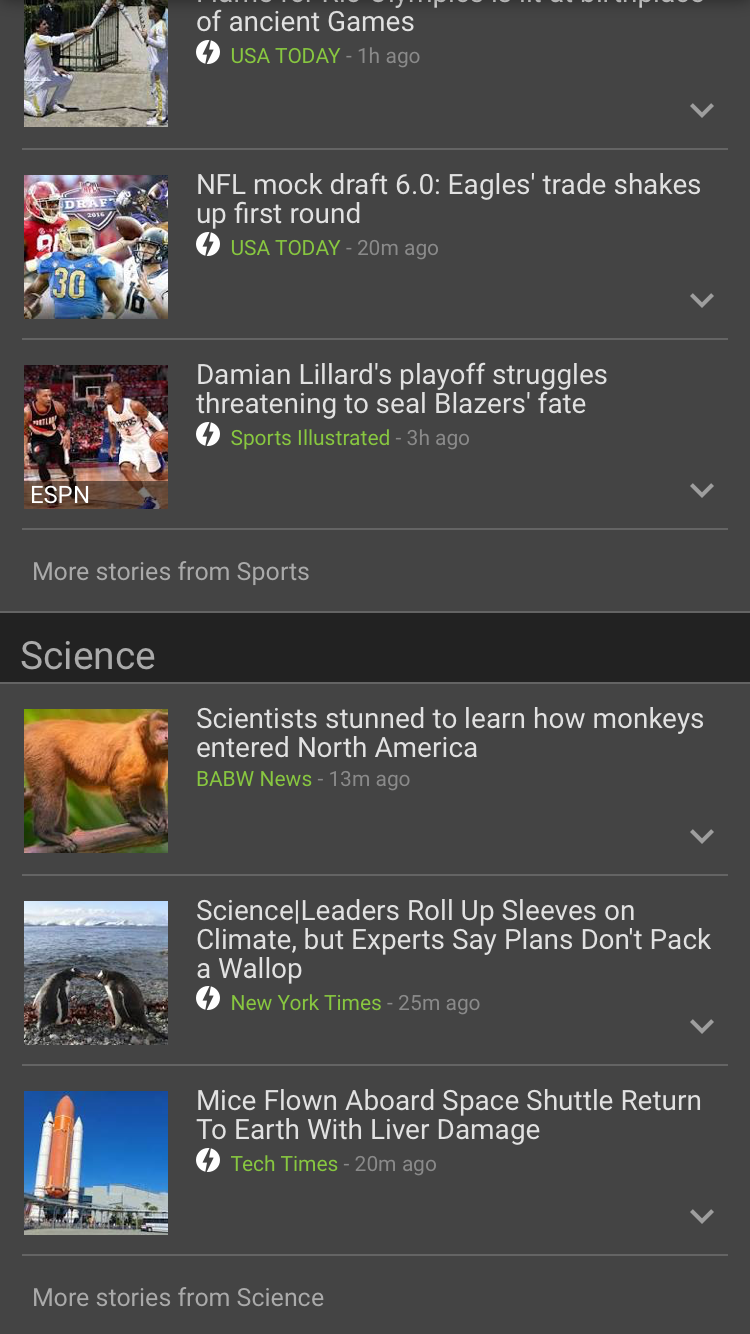This is a screenshot of a mobile device displaying a news feed with various multimedia headlines. At the top-left corner, there is an image showing two individuals dressed in long-sleeved white garments, seemingly outdoors. One person is kneeling, and they both hold long objects, possibly swords. Partly cut off to the right, the text reads, "Ancient Games," followed by "U.S. Today" with a circular logo featuring a lightning bolt. Further right, it states "An Hour Ago," along with a drop-down arrow. Below this, a second image appears, depicting football players, accompanied by the headline, "NFL Mock Draft 6.0: Eagle Street Shakes Up First Round," and timestamped "U.S. Today 20 Minutes Ago," also with a drop-down arrow to the right.

Further down, another image shows basketball action with the headline "Damien Lillard's Playoff Struggles Threatening to Seal Blazers' Fate," attributed to "Sports Illustrated," following the same format. Below, more stories are labeled under the sections of sports and science. Notably, a science section features an image of a monkey with the headline, "Scientists Stunned to Learn How Monkeys Entered North America," timestamped "BABW News 13 Minutes Ago," and a drop-down arrow. Following this, other science stories include "Science Leaders Roll Up Sleeves on Climate," and "Mice Flown Aboard Space Shuttle Return to Earth with Liver Damage," each accompanied by relevant images and similar formatting.